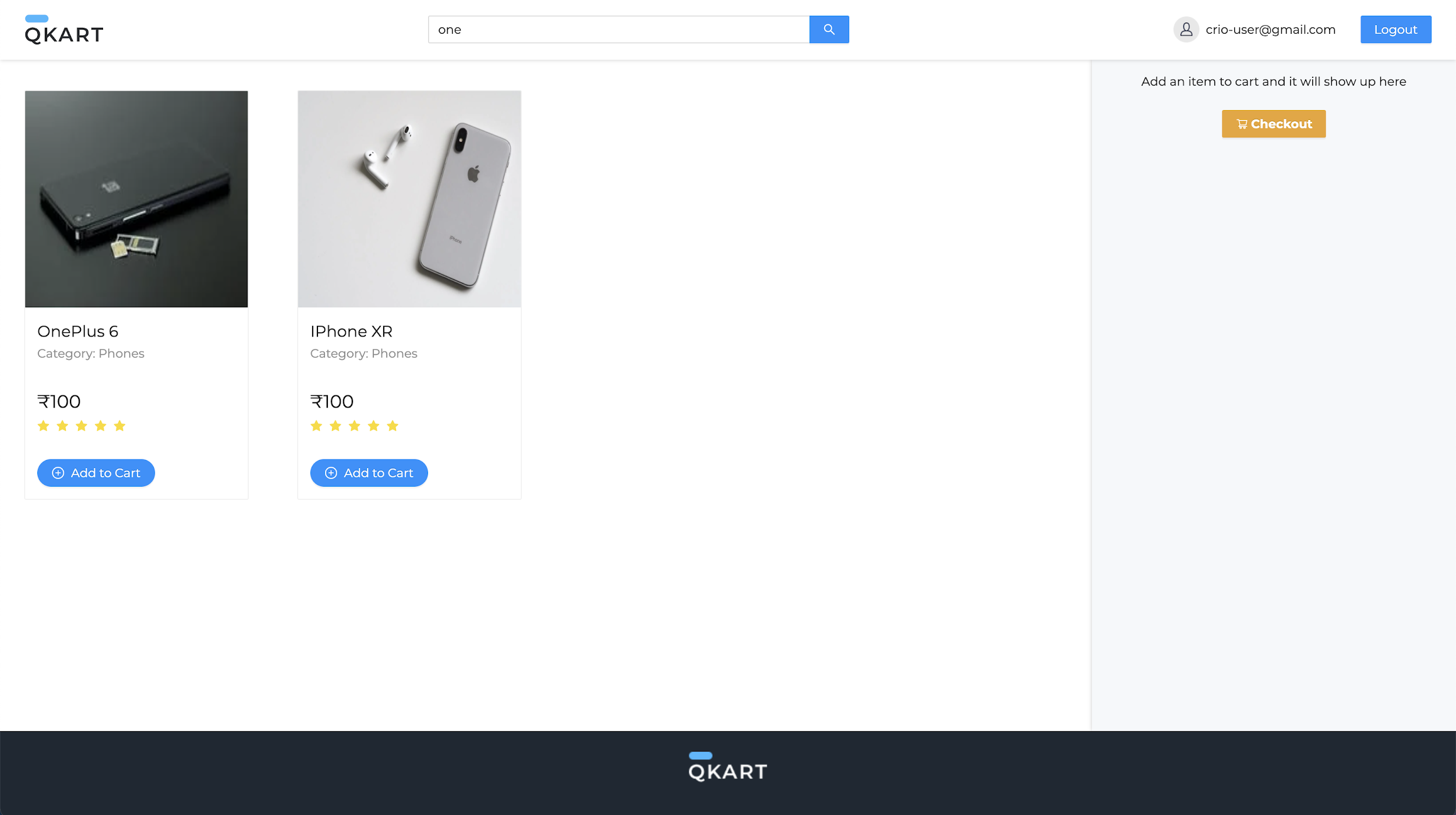This image captures a webpage from the website QCART, stylized as Q-K-A-R-T. At the very top left corner, the QCART logo is displayed in black print, featuring a short blue line over the letters 'Q' and 'K'. To the right of the logo, there's a search bar containing the text '1', and further to the right is the profile user icon. Next to the icon, the username ‘creo-user@gmail.com’ is shown, followed by a blue logout button.

The left two-thirds of the page have a white background, showcasing two product images for sale. The first product is a OnePlus 6 phone, depicted as black and placed on a dark gray background atop a black table. It boasts a five-star rating and a blue 'Add to Cart' button with white text beneath the image.

Adjacent to this, the second product on display is an iPhone XR, also carrying a five-star rating. This gray phone sits on a light gray background and a light gray table, accompanied by a pair of white earbuds. Below the image, a similar blue 'Add to Cart' button with white text is present.

The rightmost portion of the page features a light blue background. At the top, it instructs users to "Add an Item to Cart, and it will show up here" in black text. Below this, there's a brownish-yellow button with a white shopping cart icon and the word 'Checkout' in white.

At the bottom of the page, a navy blue ribbon runs across, displaying the text 'Cue Cart' in white.